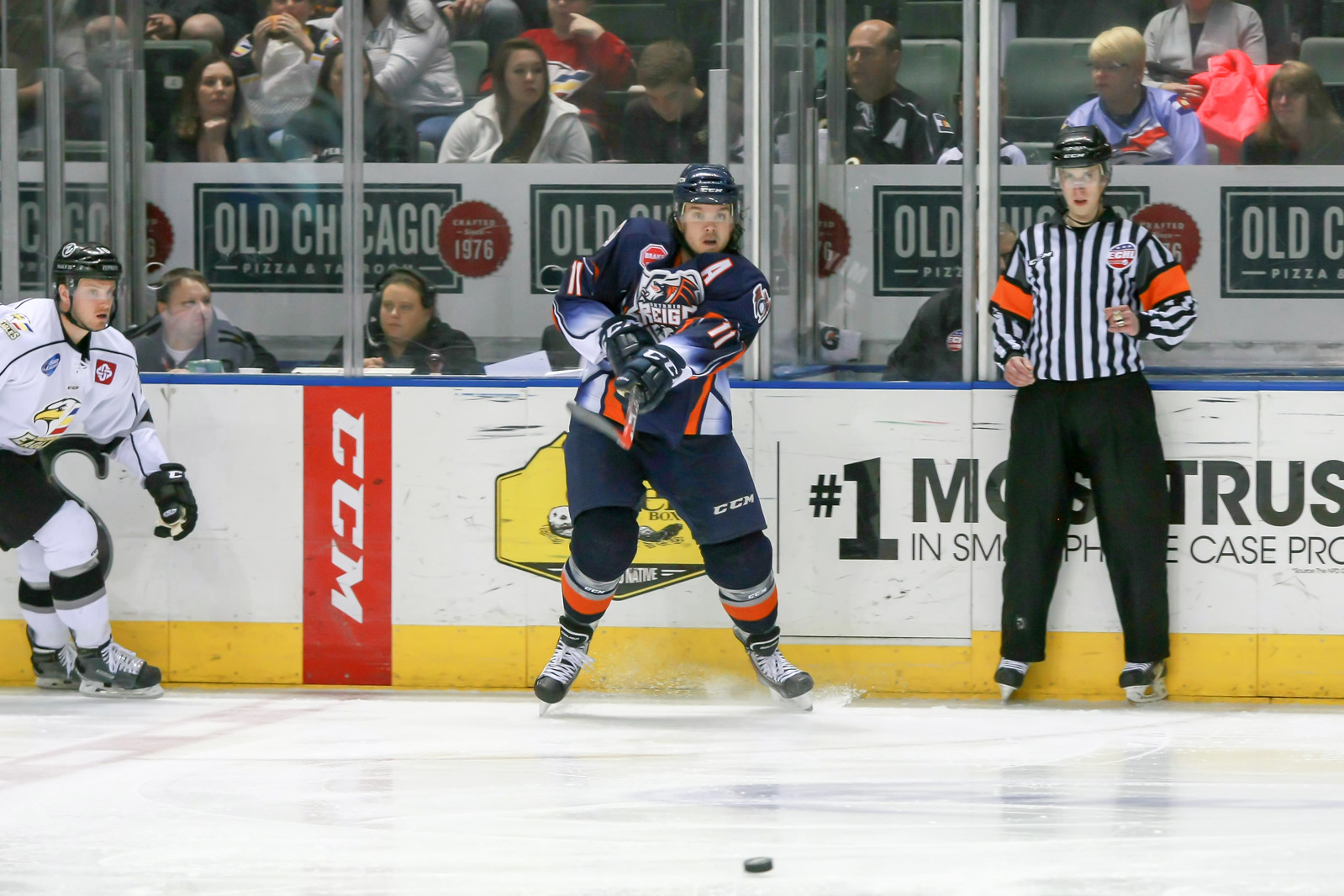This detailed image captures an intense moment in a hockey game, taken in a vibrant, bustling ice arena. At the center of the scene is a player in a dark blue and white jersey with orange pads on his legs, who is lunging forward with his stick aimed at the puck in the middle of the ice. To the left of him, an opposing player in a white uniform, black gloves, and black shorts is also moving towards the puck. On the right side of the image, the referee, clad in a black and white striped shirt with orange stripes around his arms, a protective goalie mask, and black pants, stands watching closely. In the background, behind the plexiglass, a group of officials or judges can be seen with headsets, while further back, the stands are filled with fans eagerly watching the game. Advertising signs, including one for "Old Chicago Pizza" and a sticker with "1976," add to the rich texture of the arena setting.